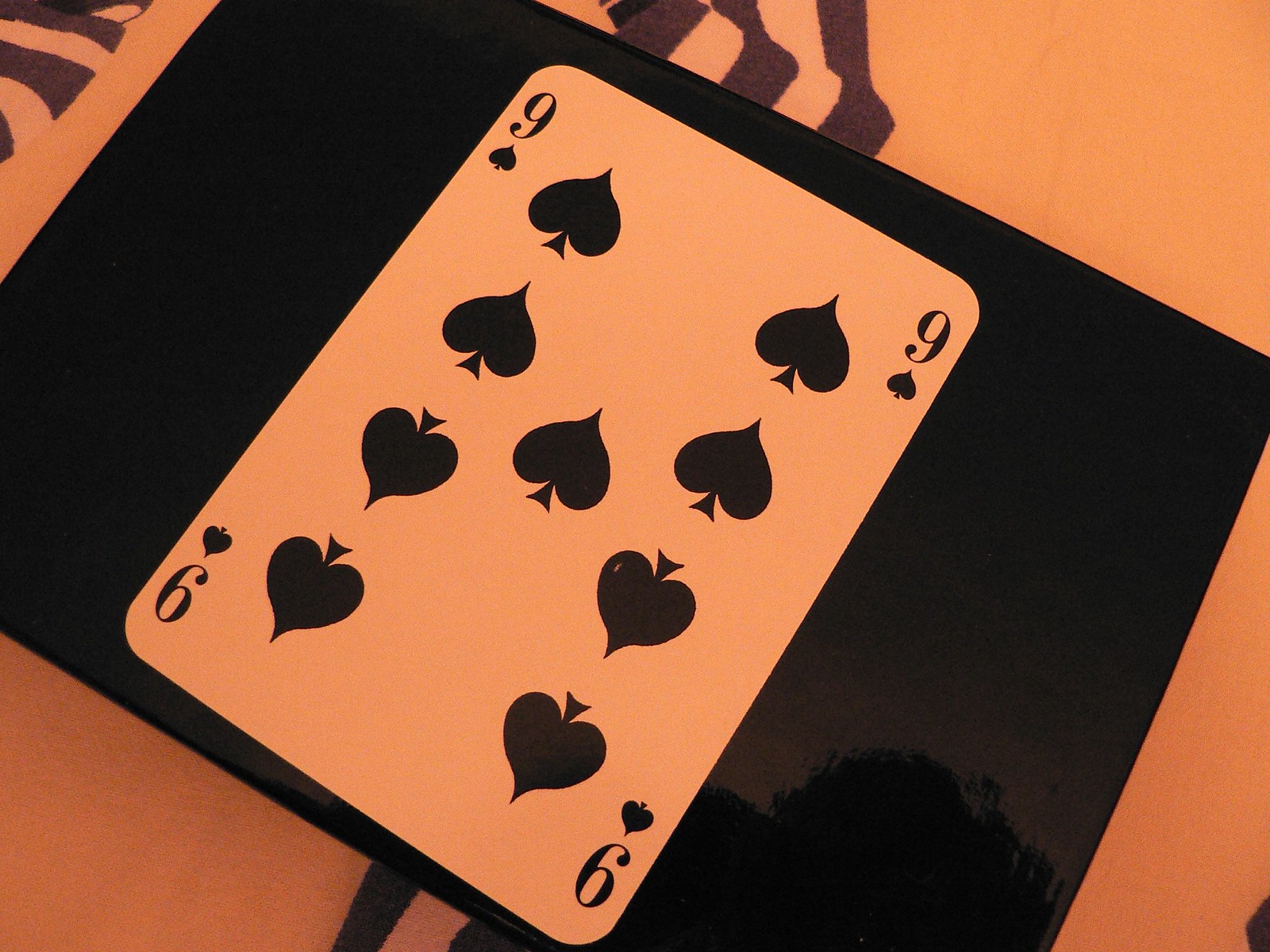The image features a playing card, specifically the nine of spades, positioned diagonally with the bottom half leaning to the left and the top half to the right. The card rests on a sleek, black reflective surface, which is slightly irregular in shape and surrounded by what appears to be a cloth or table adorned with stripe-like patterns. Notably, the picture has a distinctive filter that casts an orange tint over the areas that would typically be white while keeping the black elements true to their color. Interestingly, the reflective surface captures a partial reflection that resembles the top of a tree or a bush, adding an intriguing layer to the composition.